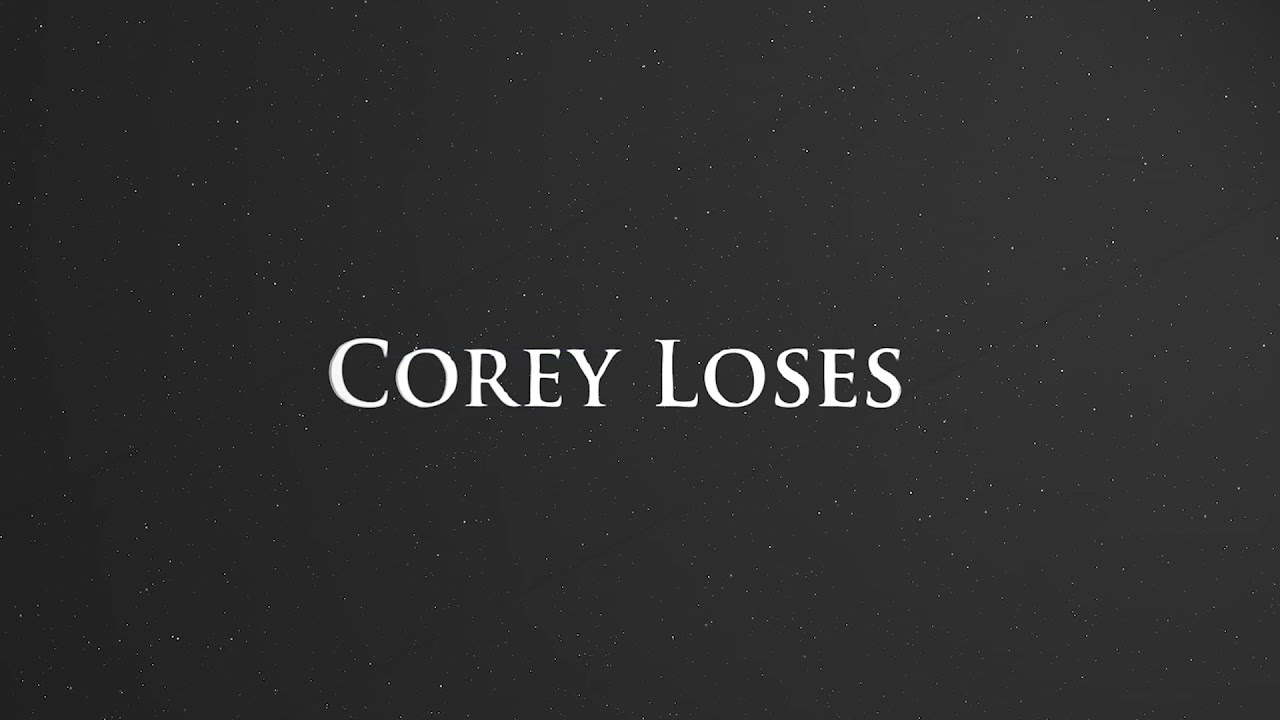The image appears to be a screenshot from a video game, characterized by a predominantly black background that mimics the appearance of a starry night sky with evenly distributed white specks resembling stars or grains of sand. The black background is split diagonally into two triangles by a faint line, adding subtle texture to the scene. Centered both horizontally and vertically in the middle of the screen, the phrase "COREY LOSES" is prominently displayed in large, white capital letters, clearly indicating that Corey, spelled C-O-R-E-Y, has lost in the game. This stark message against the dark, star-filled backdrop emphasizes the game's notification of Corey's loss.